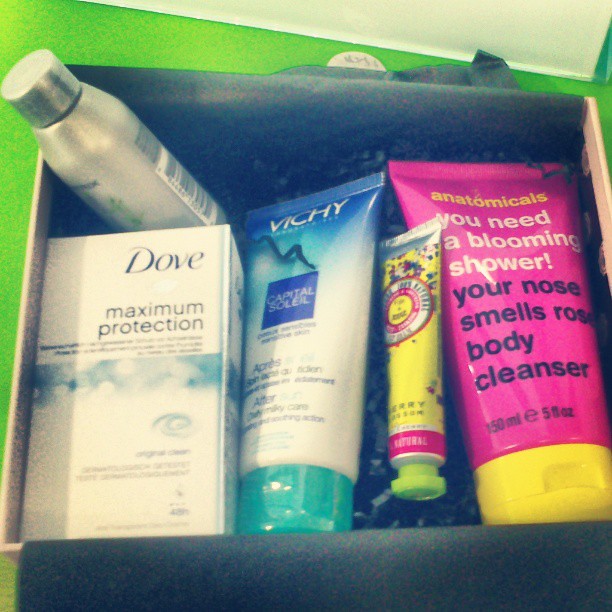This image depicts a full-color, borderless photograph featuring a cardboard box positioned on a lime-green countertop, lined with dark grey material. The box contains various skincare products. Prominently displayed on the left is a white and blue box of Dove Maximum Protection deodorant. Next to it is a squeeze-top bottle labeled "Capital Soleil," although the exact details are unclear. A small yellow tube with a green cap is also present, though the label is unreadable. Additionally, there is a pink tube with a yellow cap labeled "Anatomicals, you need a blooming shower, your nose smells rose, body cleanser." Overall, the box includes an assortment of beauty products, which appears to comprise different cleansers as well. In the background of the image, at the top, there is an indistinct white object.